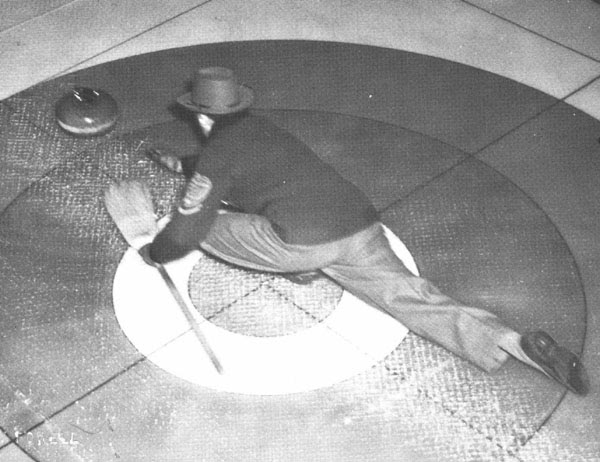This black and white photograph, likely from an earlier era, captures a man deeply engrossed in a game which appears to be curling. Positioned in a dramatic half-kneeling, half-lying posture near the center of a painted target on the playing surface, he combines determination and skill. One leg is tucked beneath his body while the other extends fully along the floor, suggesting a split-like stance. Dressed in dress slacks, black shoes, a dark-colored long-sleeved jacket, and a hat with a brim, he reaches out with his right hand toward a ceramic curling stone, resembling a pot, situated on the outer ring of the target. In his left hand, he grasps a rudimentary wooden broom, poised to influence the stone’s trajectory. The bullseye-like design of the target ground, with its concentric rings of varying shades, frames the intense moment of the sport.